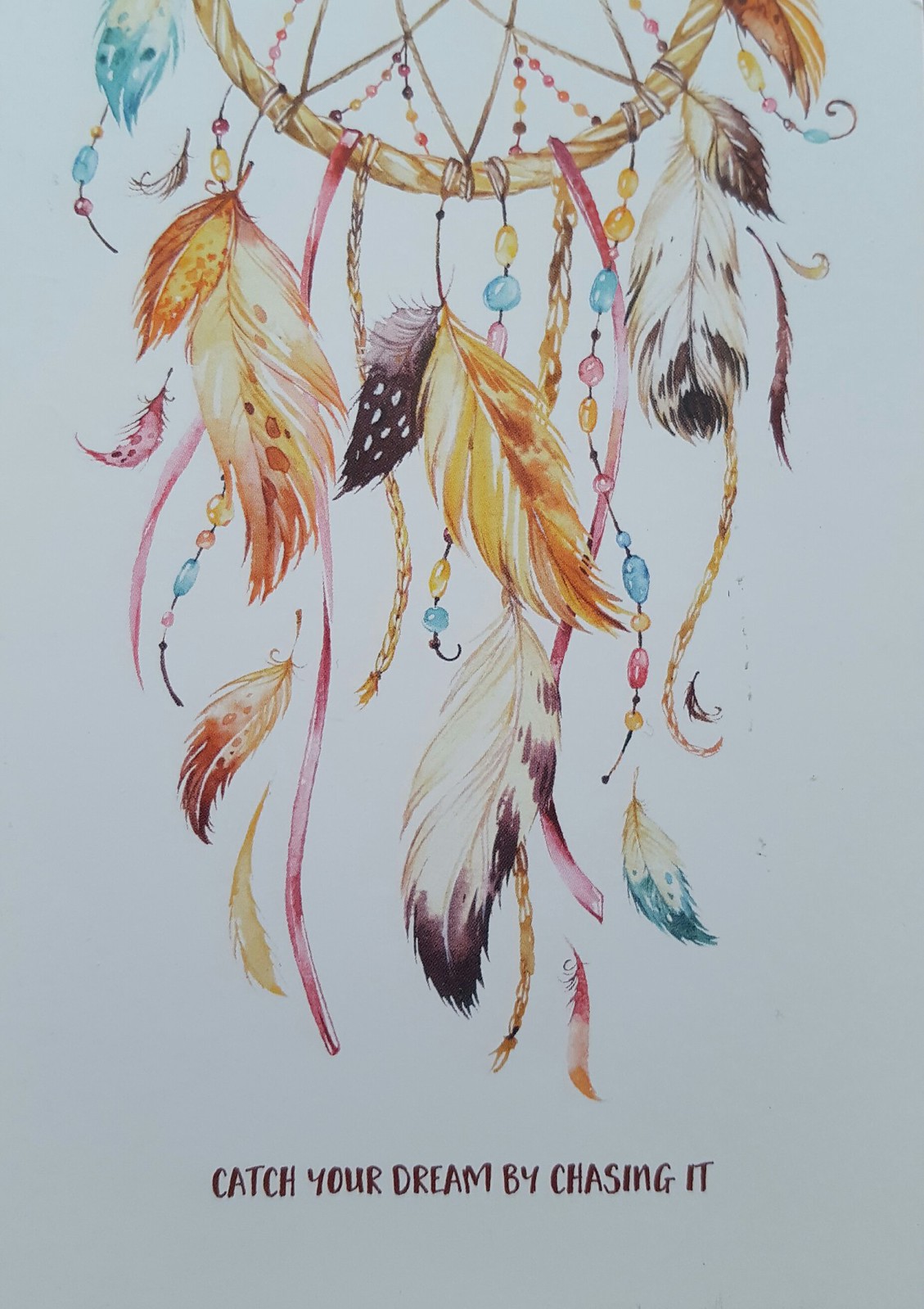The image depicts a dreamcatcher artfully positioned at the top of the frame, with only about a third of its circular portion visible. The craftsmanship is evident in the intricate design of the central web, which is adorned with assorted beads. Below the circle, an array of feathers dangle gracefully; these are a vibrant mix of orange, black and gray-mottled white, and a distinctive aqua with white highlights. Complementing the feathers, colorful beads are strung in a patterned sequence of orange, teal, and pink, varying in size. Three pink ribbons cascade down, adding an elegant touch to the composition. Prominently displayed, a title within the dreamcatcher reads, "Catch Your Dream by Chasing It," encapsulating the essence of this captivating piece.